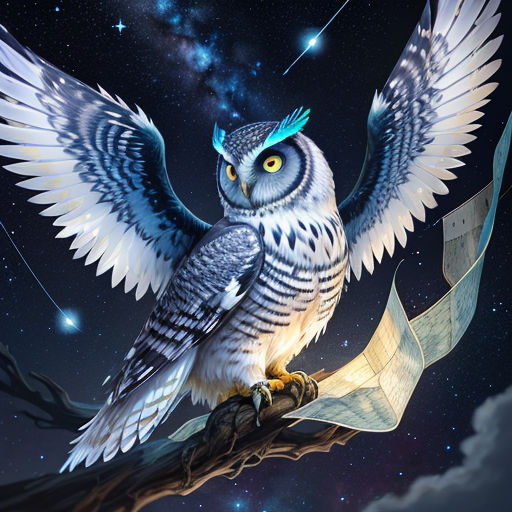This image is a detailed illustration, potentially computer-generated, depicting an owl perched on a gnarled, dark brown tree branch set against a realistic, dark blue night sky. The sky features a starry backdrop with faint white clouds near the bottom right, two blue-emitting shooting stars, and the Milky Way galaxy arcing across the scene. The owl, predominantly white with intricate black, grey, and bluish-grey feather patterns, has both sets of wings visible – one set outstretched and another folded at its sides, creating an impression of four wings. It has striking yellow eyes, a horned crest that glows teal, and bright blue feather tufts above its eyes. Clutched in its talons are long sheets of paper, possibly maps, extending from the branch. This vibrant, multi-layered portrayal blends elements of realism and fantasy, making for a captivating visual experience.